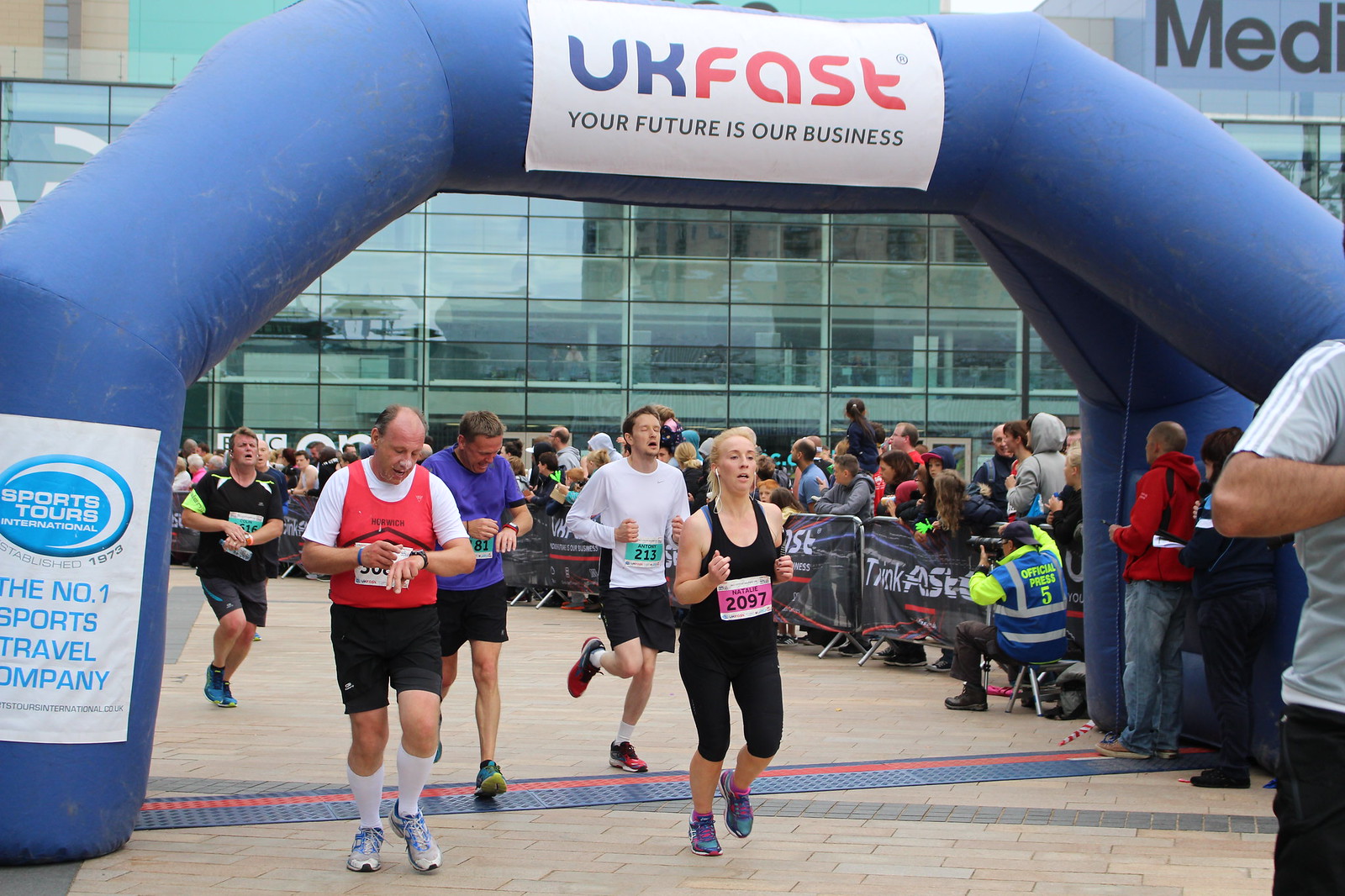This is a rectangular, horizontally aligned photograph capturing the finish line of a race, possibly a marathon or a 5K. The image prominently features a large blue inflatable archway that serves as a canopy for runners crossing the finish line. The archway displays the text "UK Fast - Your Future is Our Business" at the top, and an advertisement on the left side reads "Sports Tours - The Number One Sports Travel Company." 

In the background, there's a building with large glass windows on the lower levels, some balconies, and the partial word "MEDI" in black letters visible in the upper right corner. Several spectators are gathered behind metal barricades on the right side, cheering on the runners as they cross the finish line. 

Four runners are visible near the finish line. A woman in the lead is wearing a black, tight-fitting one-piece outfit with capris and a tank top, and a pink bib numbered 2097. To her left (our right) is a man clad in a white t-shirt with a red vest, who appears to be checking his watch; his bib number is partially obscured by his hands. Just behind them is a man in a blue shirt also checking his watch, and to his left is another runner wearing a long-sleeve white shirt with a green label indicating the bib number 213. Additional runners are seen approaching the finish line in the background, adding to the dynamic atmosphere of the scene.